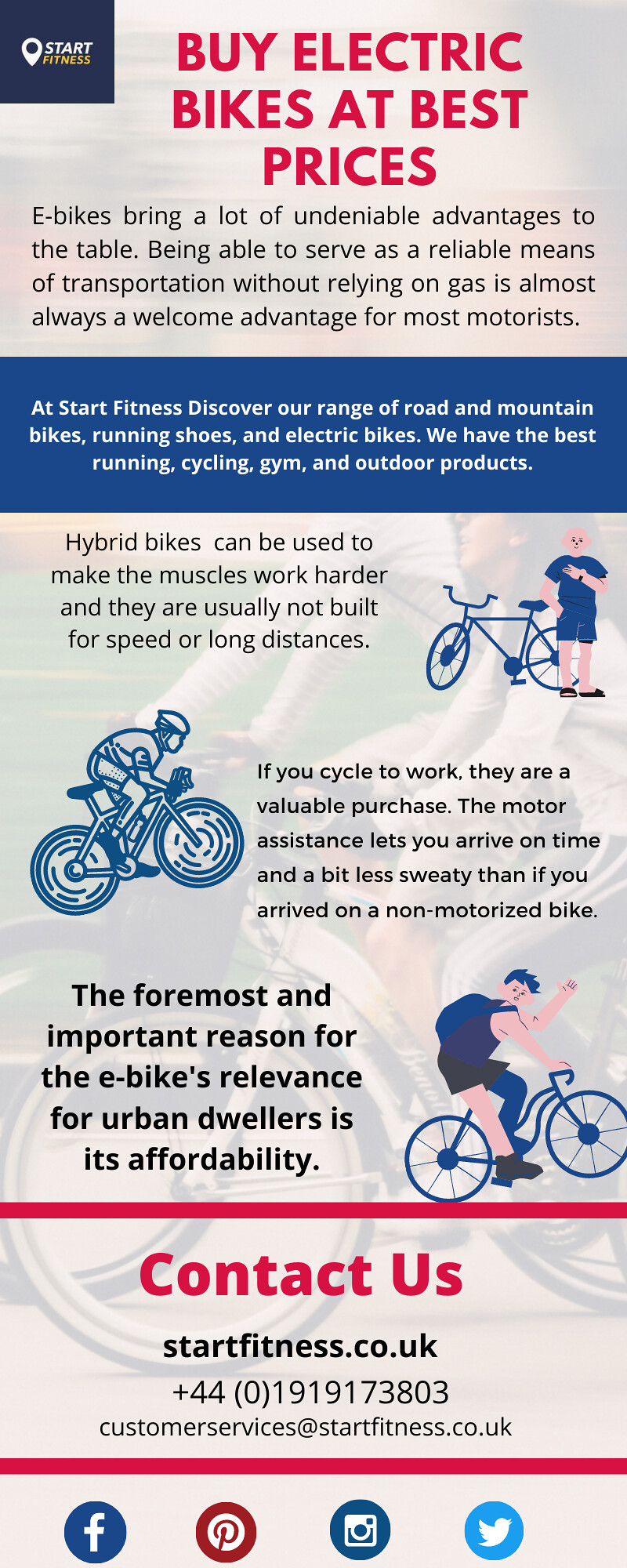This advertisement, presented in a portrait mode rectangular layout, promotes the benefits and affordability of electric bikes. At the top, striking red text reads "Buy Electric Bikes at Best Prices," followed by a black text paragraph that highlights the advantages of e-bikes, such as their reliable, gas-free operation. Directly below, a blue banner features white text mentioning Start Fitness's range of road and mountain bikes, running shoes, and other fitness products. 

The ad also includes informative sections about hybrid bikes, noting their muscle-strengthening benefits and typically slower speeds, with a cartoon illustration of a man beside a bike. Additional cartoon images of cyclists are scattered throughout the ad. An essential point emphasized is the e-bike's affordability, especially for urban dwellers, and how they make commuting more efficient and less sweaty compared to non-motorized bikes. 

Contact information for Start Fitness is provided at the bottom, including a website URL, a phone number, and an email address, all separated by a horizontal red border. The ad is concluded with icons for Facebook, Pinterest, Instagram, and Twitter, encouraging social media engagement.